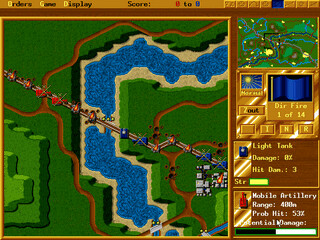In this rectangular screenshot from a vintage video game, the graphics are simple and not very high-tech. The screen showcases a game environment with a green square patch of land, intersected by a bright blue, crescent-shaped body of water that is edged with beige areas, likely representing sandy beaches. The user interface includes text elements against an orange background at the upper left corner, displaying categories such as "Orders," "Display," and "Score" in sequence. On the lower right corner, text descriptors provide detailed information about a unit named "Mobile Artillery," including statistics like "Artillery Range: 400," "Probability of Hit: 53%," and "Damage." The image is not high-resolution, reflecting the vintage nature of the game.